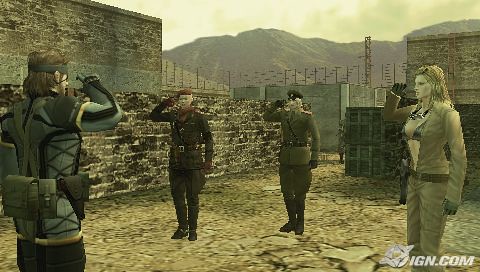The image appears to be from a computer game, depicting a scene with four characters engaged in a salute. In the foreground, there is a male figure shown from the back. He is equipped with a belt loaded with various items, including what seems to be a holster. Facing this figure are three other characters. One of them appears to be a woman, identifiable by her long blonde hair. She is dressed in coveralls that are open at the waist, exposing part of her outfit underneath. The second character gives the impression of a World War II-era German Nazi officer, complete with the uniform. The third character's gender is ambiguous, but they seem to have a similar German military appearance. The backdrop features a courtyard setting with stone steps, surrounded by buildings and fencing. In the far distance, mountains enrich the scene, adding a sense of depth and context to the environment.